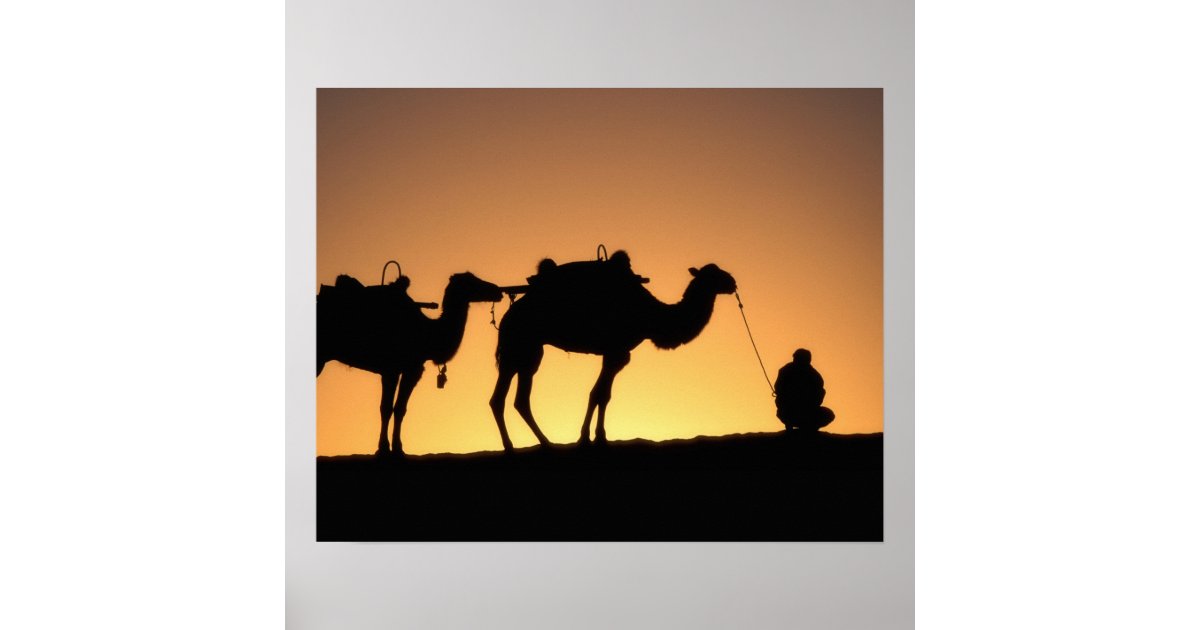The image depicts a striking silhouette scene at either sunset or sunrise. Two camels, both with saddles and connected by leashes, stand in a line facing towards the right. The first camel is fully within the frame, while only the hind legs of the second camel are visible on the left side. To the right, a man squats on the balls of his feet, holding one of the leashes. All the figures—the man, the camels, and the land they stand on—are rendered in stark black silhouette against the vibrant background. The sun, positioned near the horizon, emits a radiant glow, transitioning from a brilliant yellow to a warm orange, casting an enchanting light over the desert landscape.